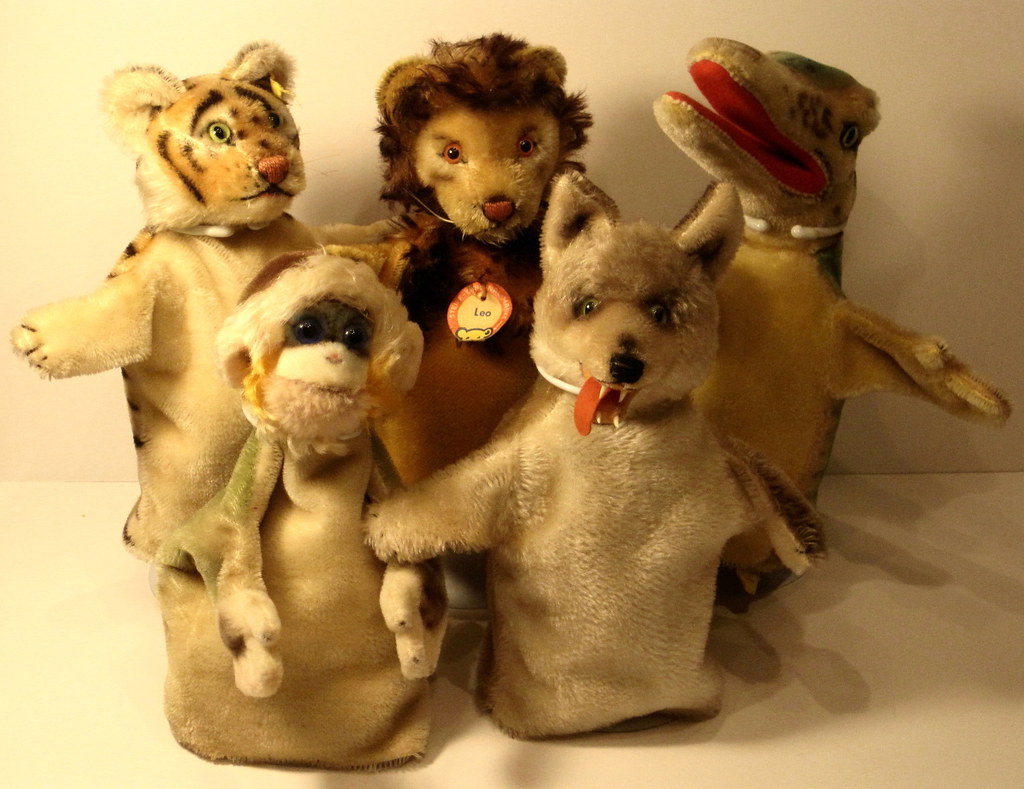This image depicts five vintage animal-themed hand puppets, arranged in a row and seated upright on a table, with no hands inside them. From left to right, the puppets are a tiger, a lion, a crocodile, a wolf, and a monkey. The puppets show signs of age, with their colors looking faded and worn.

The tiger on the far left is light orange with black stripes, green glass eyes, a pink nose, and an outstretched arm. Adjacent to the tiger is a lion, softly beige with a darker brown mane, yellow eyes, and a pink nose. It is the only puppet with a circular collar tag reading "Leo."

Next is the crocodile, light green with a yellowish belly, noticeable teeth inside its wide red mouth, and a white brace around its neck. In front of the crocodile sits the wolf, which is gray with a red tongue sticking out of its mouth, sharp pointy teeth, and short, stubby hands.

The monkey, positioned closest to the camera, is light brown with little black eyes and small yellow tufts on either side of its cheeks. It features some worn greenish fur on its back. All the puppets have short, stubby hands, adding to their vintage charm.